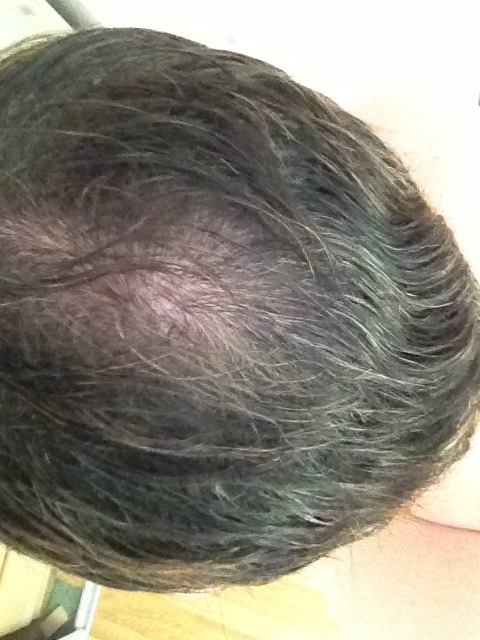This photograph, measuring approximately 5 by 7 inches, depicts the top of a man's head, which occupies the center frame. The man, experiencing male pattern baldness, has salt and pepper hair that is a couple of inches long. The image focuses on his head, but a glimpse of his shoulder is visible, suggesting he might be wearing a white shirt or apron, possibly indicating a setting like a barbershop. The background includes detailed elements such as a green and yellow wooden floor and indistinct objects, possibly tools or boxes, in the bottom left corner. The image is slightly unclear, with additional elements like a white area in the top right and possibly a line or pole in the top left, adding to the setting's indoor feel. Notably, the photograph contains no text, date, or identifying information.